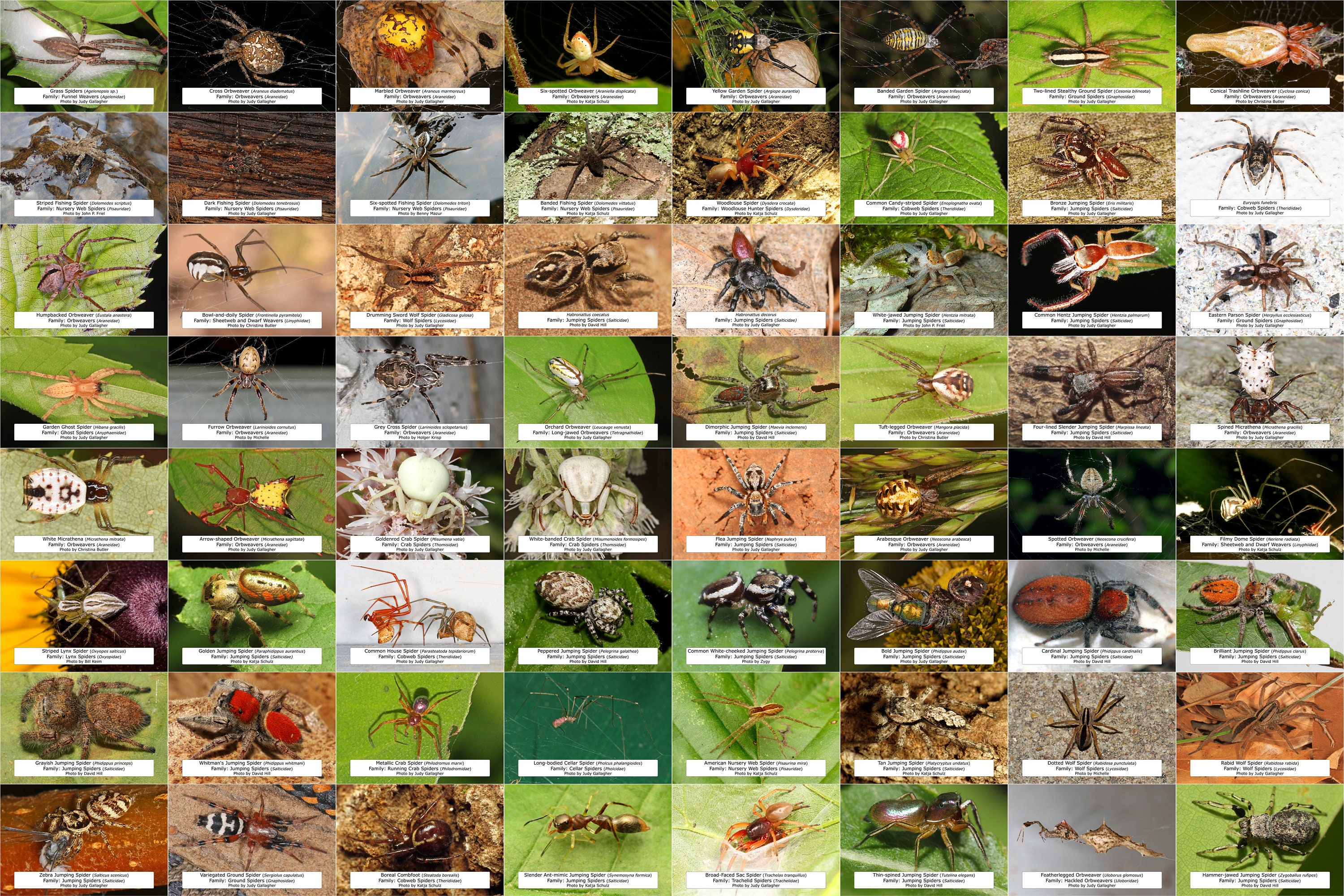This is a detailed caption for an image of a poster:

The image depicts a large, horizontally rectangular poster featuring 64 vividly colored photographs of various spiders, predominantly orb weavers, jumping spiders, and wolf spiders. The poster is organized into a grid with eight rows and eight columns, showcasing spiders in their natural habitats, mostly on leaves or the ground. Each spider has a distinct appearance, with some having stripes, polka dots, or striking colors such as black, yellow, and red. Underneath each spider's photograph is a long white rectangle containing black text, presumably naming or describing the species. The layout and identical labeling areas suggest it's professionally made rather than an online collage. Alongside the numerous spider images, there are also a few insects, including a bee and an ant, adding to the diversity of this entomological collection.